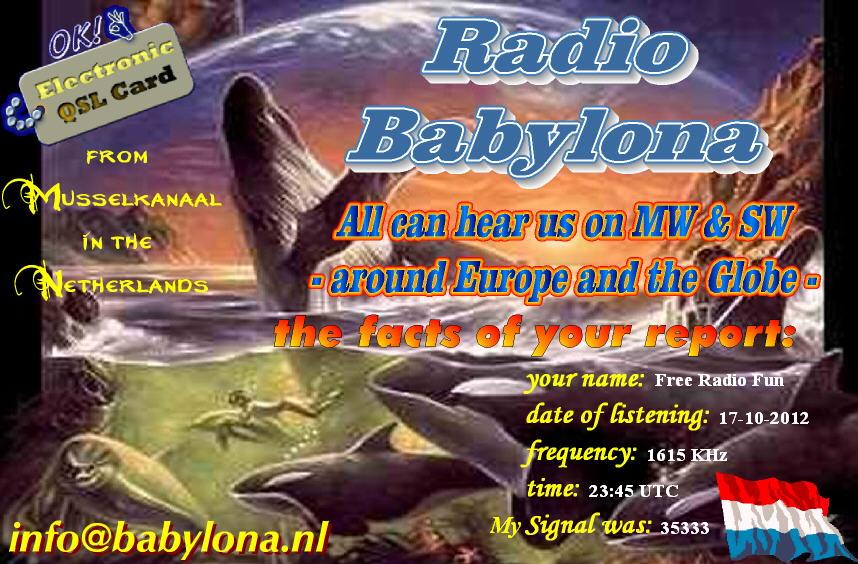This is a detailed promotional image for Radio Babylonia set against a vivid, artistic background depicting a rich marine scene. The illustration features vibrant sea life including whales and dolphins jumping out of the ocean, alongside children swimming. The scene is bathed in hues of purple, green, and sunset colors, with a moon and rocky formations adding to the atmosphere. On the left side, there's text indicating "Electronic SL Card from Mussel Kanaal in the Netherlands." On the right-hand side, further text reads: "Radio Babylona: All you can hear us on MW and SW around Europe and the globe. The facts of your report: your name, free radio fun, date of listening 17-10-2012, frequency 1615 KHZ, time 23:45 UTC, signal 35333. For more information, visit info@babelona.nl." A Dutch flag waves in the lower right corner with red, white, and blue horizontal stripes.